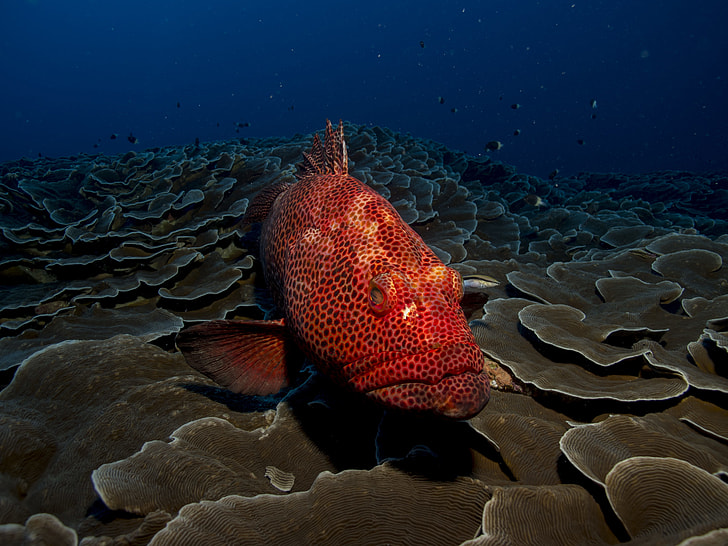Captured in an underwater scene, this vibrant photograph reveals the mesmerizing world beneath the ocean's surface. The ocean floor is blanketed with an intricate tapestry of dark, cabbage-like plants, each leaf a deep black with delicate blue outlines and crisscrossed with fine lines, resembling giant black lily pads stacked in multiple layers, creating a surreal underwater landscape.

At the heart of this captivating scene is a striking red fish, adorned with a pattern of black and white spots. Its prominent eyes are encased in bulging sockets, and it features distinctive, fleshy fish lips. The fish faces the camera directly with a closed mouth, showcasing its impressive fins that transition in color from red to dark red, tipped elegantly in black. Noticeable along its back are pronounced spikes, adding to the fish's intriguing appearance. The perspective of the photograph, tilted slightly, also includes other smaller fish in the background, though they are somewhat obscured by the angle and distance. The main fish dominates the scene, with its left side most prominently visible, providing an intimate glimpse into its underwater existence.